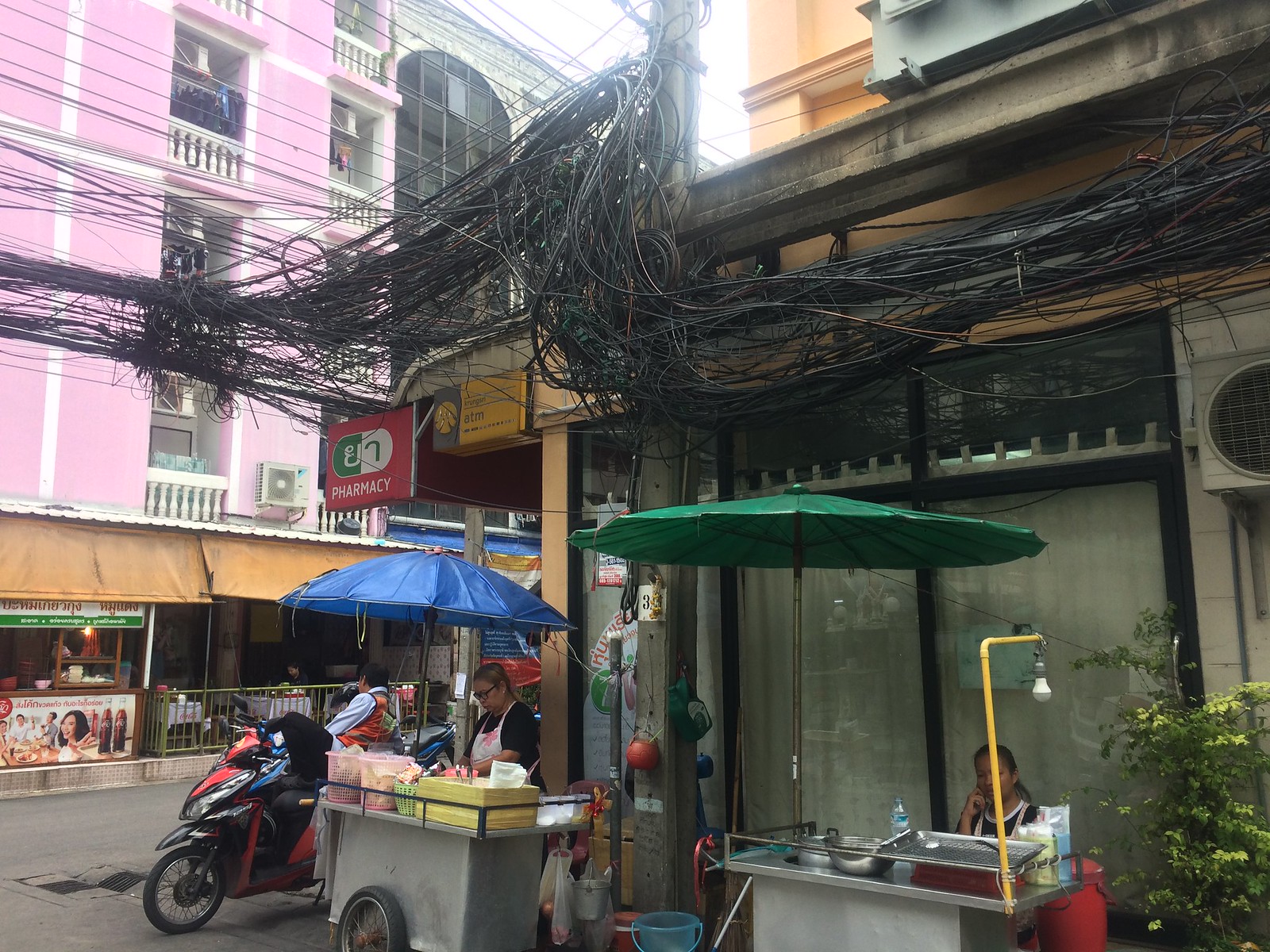This photograph, taken in a bustling Southeast Asian city—possibly Thailand or Vietnam—captures a vivid street scene rich with details. Dominating the view are the tangled, dense clusters of electrical wires stretching from a utility pole across the street to various buildings, reminiscent of Bangkok or other urban areas in the region. Below this chaotic web of cables, street vendors set up their carts along the sidewalk. In front of a shop front building with split-unit air conditioning units, two women manage their food carts. The older-style hotel or commercial building on the right boasts a large AC unit and balconies with white wooden railings, alongside colorful storefronts and awnings beneath. One vendor sits behind a metal cart equipped with a green umbrella, two metal pots, and a silver pan, while another vendor stands, wearing an apron, beside her cart that features pink bins and a wooden box, and is shaded by a bright blue umbrella. Nearby, a motorcycle and scooter are parked, indicative of the localized modes of transport. Coca-Cola advertisements add a splash of commercial familiarity to the vibrant streetlife, with an intersection visible in the distance, further enhancing the dynamic urban atmosphere.